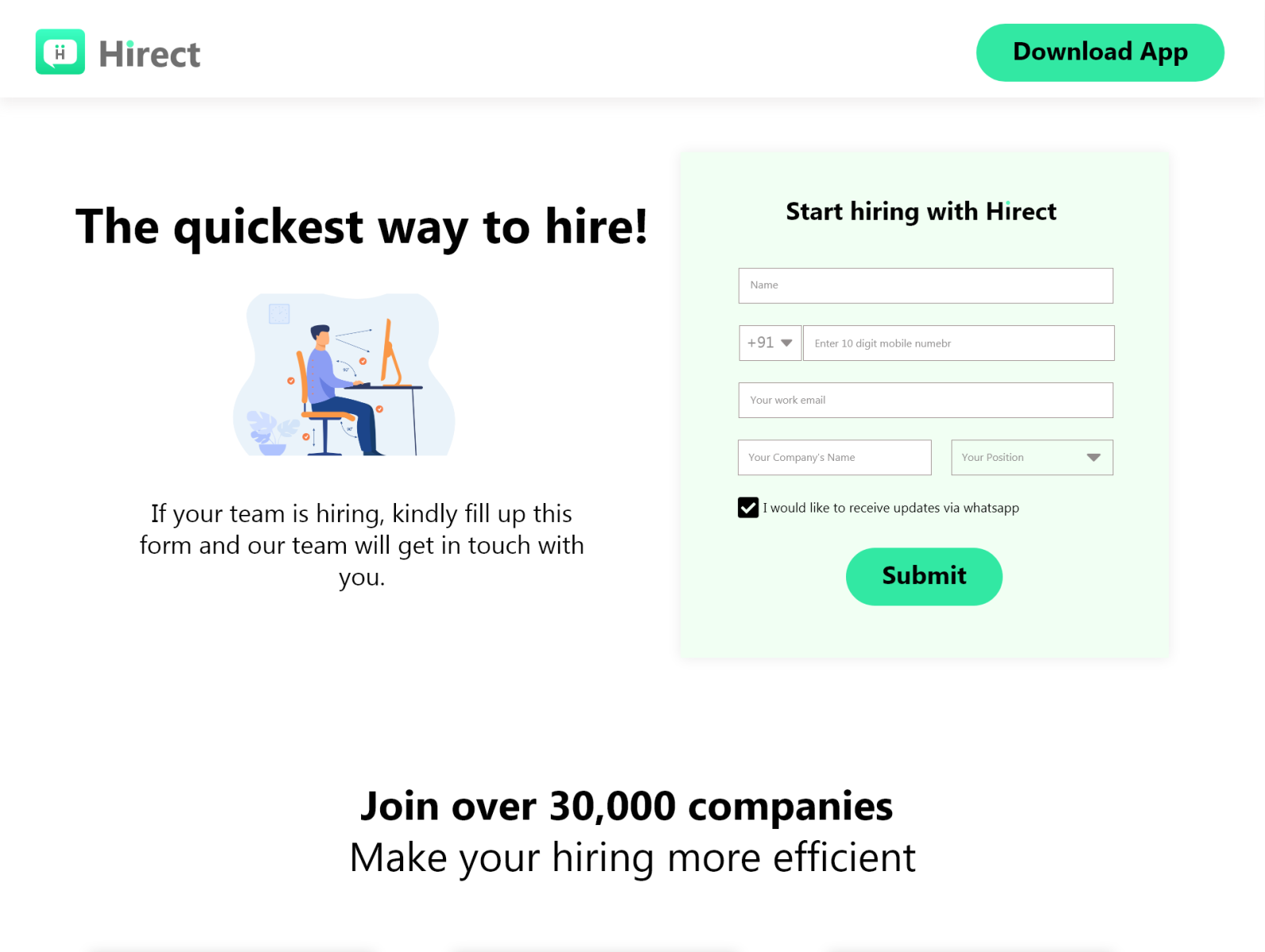The image depicts a desktop screenshot, missing visible elements of the browser, link, or operating system. In the top left corner, there is a green square icon featuring a white chat bubble with two green dots and an "H." Adjacent to this icon, "HIRECT" is written in black text with a green dot replacing the "i." 

To the right, there is a light green, pill-shaped button labeled "Download App." Right beside it, the phrase "The quickest way to hire" is displayed. Below this, a cartoon illustration portrays a man with dark hair, dressed in a blue sweater and darker blue pants, sitting at a desk on an orange chair in front of an orange computer, surrounded by whimsical swirly animations.

The text on the image encourages teams that are hiring to fill out a form to be contacted by the HIRECT team. To the right, another message reads, "Start hiring with HIRECT," accompanied by fields to input a name, select a country code, enter a mobile number, work email, company name, and position. There is also a checked checkbox that states, "I would like to receive updates via WhatsApp." Below this, a green pill-shaped button with black text invites users to "Submit."

At the bottom of the image, a call to action reads, "Join over 30,000 companies, making your hiring more efficient." This detailed setup suggests that HIRECT is an app designed to facilitate the hiring process efficiently.